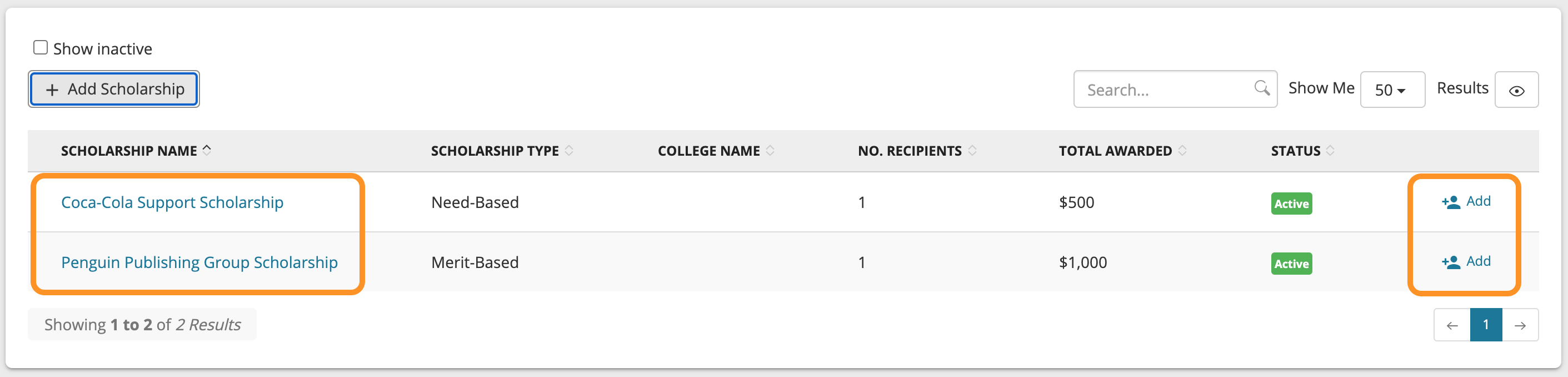The image is a detailed and compact representation of a scholarship tracking interface, laid out in a long horizontal rectangular format with a predominantly white background. 

**Top Section:**
- **Top-Left:** A light gray outline of a checkbox.
- **Right of Checkbox:** Black text stating "Show inactive".

**Main Interface:**
- **First Row beneath Top-Left:** A light gray rectangular box housing light gray text that reads "Add Scholarship", accompanied by a plus sign on the left of the text.
- **Second Row (Spanning the Width):** A series of aligned categories within a long light gray rectangular box:
  - **Leftmost**: "Scholarship Name" in black text.
  - **To the right:** "Scholarship Type" in black text.
  - **Next:** "College Name" in black text.
  - **Next:** "No. Recipients" in black text.
  - **Next:** "Total Awarded" in black text.
  - **Rightmost:** "Status" in black text.

**Search and Filter Options:**
- **Above "Total Awarded" Column:**
  - A rounded-edged search bar.
  - Adjacent to the search bar: Black text reading "Show me".
  - Followed by a small rectangular box containing the number "50".
  - "Results" in black text.
  - Another small rectangular box to the far right.

**Scholarship Listings (Two Rows):**
- **First Row (Scholarship Details):**
  - **Leftmost in Blue Text**: "Coca-Cola Support Scholarship".
    - *Under "Scholarship Type":* "Need-Based".
    - *Under "No. Recipients":* "1".
    - *Under "Total Awarded":* "$500".
    - *Under "Status":* "Active".
- **Second Row (Scholarship Details):**
  - **Leftmost in Blue Text**: "Penguin Publishing Group Scholarship".
    - *Under "Scholarship Type":* "Merit-Based".
    - *Under "No. Recipients":* "1".
    - *Under "Total Awarded":* "$1,000".
    - *Under "Status":* "Active".

**Far Right of Each Row:** 
- Blue text labeled "Add" for additional actions.

The meticulous layout aids in navigating scholarship information efficiently, showcasing each scholarship's type, recipients, award amounts, and status in an organized and approachable manner.